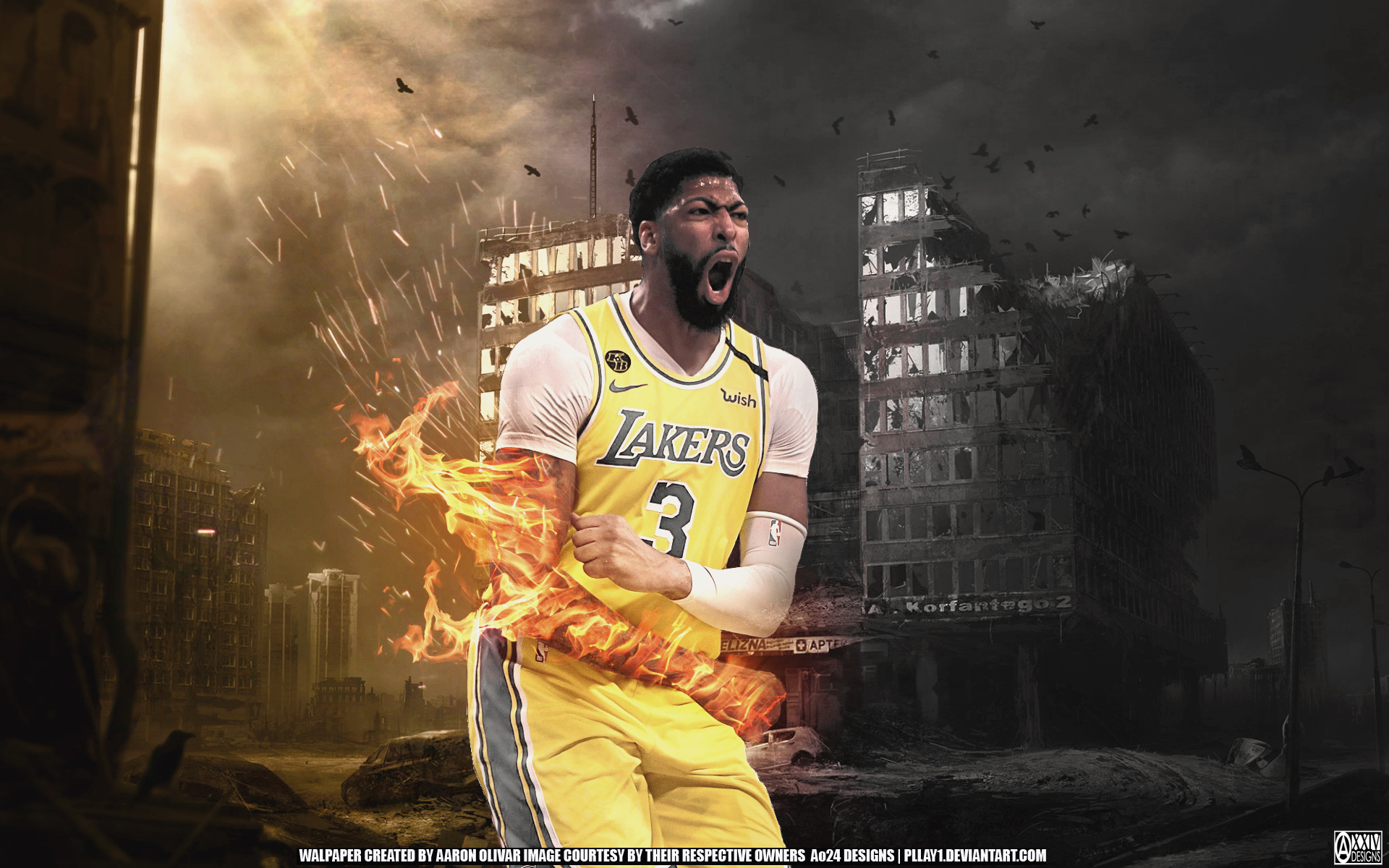The image features basketball star Anthony Davis prominently in the center, dressed in his yellow Lakers jersey with purple text displaying "Lakers" and the number 3. One of Davis's arms is engulfed in flames, while the other is normal, donned with a white arm sleeve. He is captured in a moment of intensity, possibly yelling. The background portrays a ravaged, apocalyptic cityscape with deteriorating and partially destroyed buildings. The smoky sky adds to the desolate atmosphere, with faint rays from the sun peeking through at the top left. The color palette includes yellow, blue, purple, gold, flame yellow, flame orange, black, white, several shades of brown, and beige. At the bottom of the image, text in white credits the wallpaper creation to Aaron Olivar, with the image courtesy of AO24designs and PLAY1.deviantart.com.